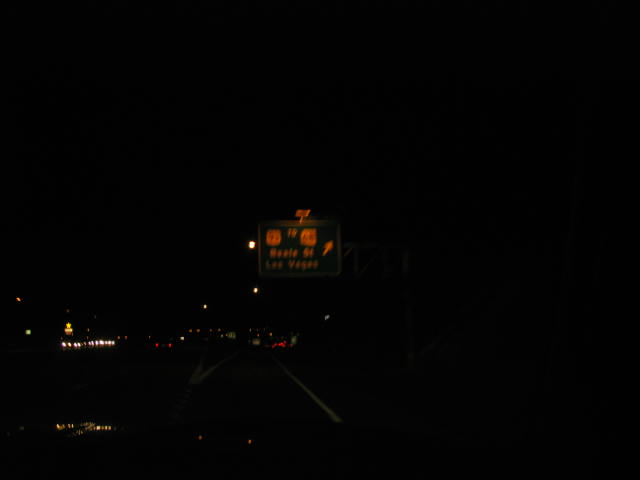In this very dark nighttime photograph, the scene captures a stretch of highway. The sky and background are almost entirely black, casting an overall dim atmosphere. On the left side, you can discern the interior of a car, including dimly lit dashboard lights, suggesting the photo was taken from within the vehicle. The road ahead reveals various features: white lane lines and a green exit sign marked for Las Vegas with a white arrow. 

Several lights are visible in the distance, including red brake lights of cars traveling away from the camera and white headlights from oncoming vehicles. Along the roadside, there are sporadically lit streetlights, and some illuminated signs from nearby buildings can also be noticed. The image also includes orange lights that resemble pumpkins, possibly from Halloween decorations or simply reflections. The far-off lights are mirrored on what appears to be a water body below, adding a subtle glow to the dark surroundings. The majority of the right side of the photo remains in deep shadow, preserving the night’s obscurity.